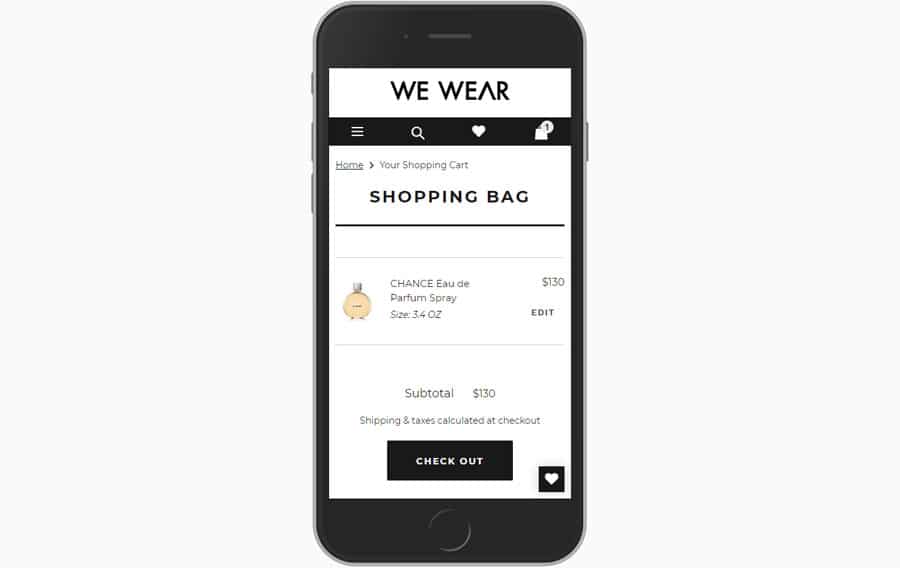The image is a square graphic featuring a black smartphone. The phone's screen displays a shopping interface with several icons and elements. At the top, there's a black navigation bar with a slightly distorted brand logo where the 'A' is missing the horizontal line. 

The header includes four white icons: a hamburger menu, a magnifying glass, a heart, and a shopping bag with a number '1' in a circle indicating one item in the cart. 

Below the header, the interface shows a navigation menu with labeled tabs: "Home," "Your Shopping Cart," and "Shopping Bag." 

The main content area displays a product listing for a perfume. There is an image of a spray bottle labeled "Chance Eau de Parfum Spray, Size: 3.4 ounces." 

The listed price for the perfume is $130. Towards the bottom, there is a subtotal listed as $130 with a note indicating that shipping and taxes are calculated at checkout. Next to this is a black rectangular button labeled "Checkout."

Adjacent to this, there is another black square containing an image of a hamburger adorned with a white heart icon.